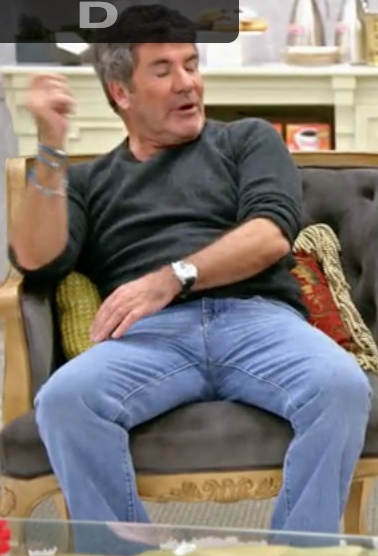The image depicts a man, who resembles Simon Cowell, sitting in a deep black fabric chair with a light wooden frame. He is relaxed and leaning back slightly, with his head turned to the right, eyes closed, and mouth slightly open. He is dressed in blue jeans and a long-sleeved black shirt with the sleeves rolled up above his elbows. On his right wrist, he wears multiple blue bracelets, and on his left wrist, he has a prominent silver wristwatch.

In the foreground, there is a glass-topped coffee table that obscures the view of his feet. The chair features a vibrant red pillow with yellow frills positioned behind him and a yellow and green plaid pillow to his left side. 

Behind the man, a fireplace filled with boxes of unopened coffee is visible, alongside various items placed on the mantel. The scene is accentuated by homey yet cluttered surroundings, giving an impression of a cozy but lively living area.